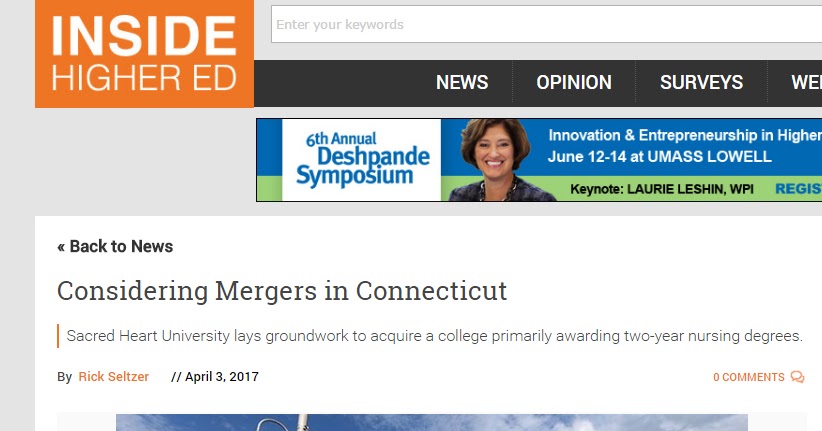The webpage depicted appears to be a news or opinion platform, possibly focused on higher education. In the top left corner, an orange box displays the title "Inside Higher ED," suggesting that this site caters to higher education topics. Adjacent to the title on the right is a search bar. Below this, a black banner lists various sections including "News," "Opinions," and "Surveys," though some text is truncated and unclear.

Following this navigation bar, there is an advertisement featuring a "6th Annual Deshpande Symposium" along with an image of a person, indicating a promotional banner for an educational symposium or learning event. Directly under the advertisement, a link titled "Back to News" is visible. Beneath this, a news article headline reads, "Considering Mergers in Connecticut: Sacred Heart University lays groundwork to acquire a college primarily awarding 2-year nursing degrees," authored by Rick Seltzer and dated April 3rd, 2017, with zero comments at the time.

An article begins just below this headline, accompanied by a partially visible image that seems relevant to the news story. The overall background of the webpage is predominantly white, with some gray areas near the top where the banners are located.